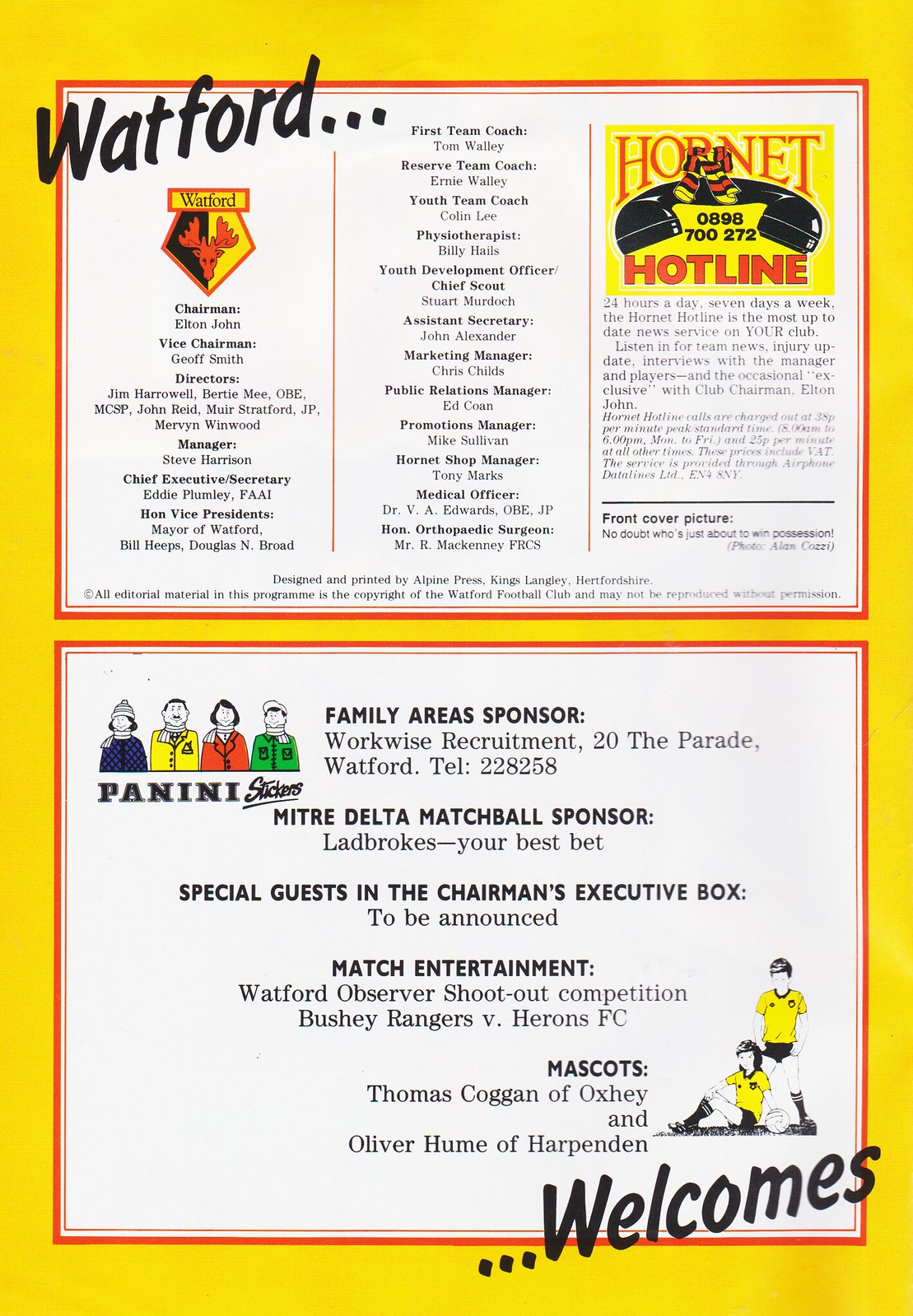This image is a detailed scan of a program page for Watford Football Club, set against an orange background. The page is divided into two primary sections, both outlined in red. The upper section prominently features the word "Watford" in stylized print with three dots leading the viewer's eye. To the top left, it includes the club’s crest—a yellow rectangle with the name "Watford," and within a red outlined shape resembling the head of a pen, is a red reindeer figure. Below this, the list of key figures is enumerated, commencing with the “Chairman: Elton John.” On the right of this section, a yellow box with an old-fashioned phone receiver icon highlights the "Hornet Hotline" and the number listed as 0898 700 272. This section underscores the organization’s leadership and a hotline for club inquiries.

The lower section of the program features content linked to the club's activities and sponsors. On the left, an illustration depicts four figures in differently colored coats—blue, yellow, red, and green—likely representing the "Pennelly stickers" advertisement. Below this, text announces various sponsorships and event details, such as "family areas sponsor: Work-Wise Recruitment" along with the address, and contributions from Ladbrokes for the MITRE Delta match ball. Additional highlights include a "Watford Observer Shootout Competition" between the Bushy Rangers and Herons FC, and the notation of special guests to be announced in the "Chairman's Executive Box." The mascots, Thomas Goggin of Oxley and Oliver Hume of Harpenden, are also mentioned.

Finally, the page concludes with warm welcomes, using a font consistent with the initial "Watford" header. Two young individuals in yellow tops are depicted in the right-hand corner, enhancing the community and familial atmosphere promoted by the club.